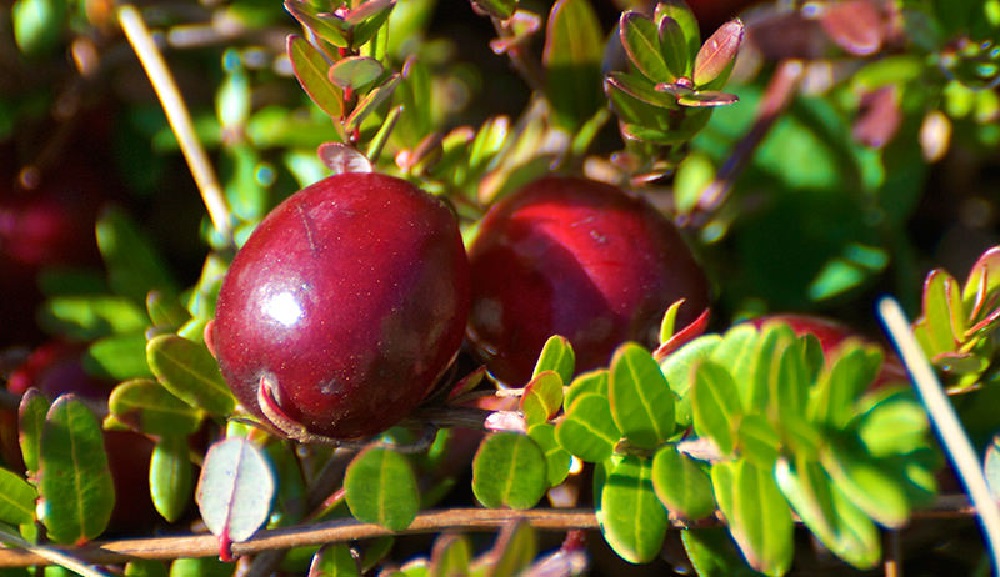The image is a close-up of a shrub displaying several large, round, smooth red berries prominently in the center. The berries, resembling grapes, are vividly red with a few white dots, and the one to the left center has a noticeable shiny spot and even a scratch. In contrast, the berries further back are blurred out. The plant features thin branches with small green leaves, some edged or centered with red, a few of which have a distinct yellow line bisecting them, while the ones at the bottom right show a slight purplish sheen. There appear to be larger leaves from a different plant in the shadowy background, which is also blurred, bringing more emphasis to the well-lit front. The branches seem to be tied to something artificial to keep them upright.